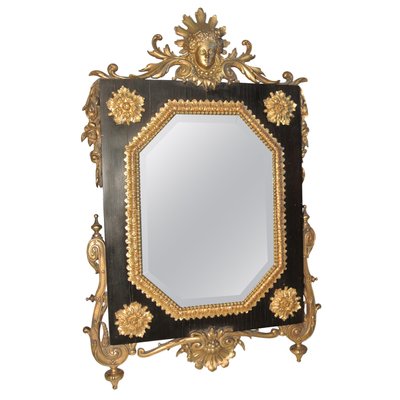This image displays an antique, ornate mirror with an elaborate gold frame set against a white background. The top of the mirror features an intricate design showcasing an angel's face adorned with a headdress, alongside scrolling foliage patterns and leaves that extend downward along the sides. The bottom of the frame echoes this leaf motif, wrapping around the base, and is intricately detailed with a complementary pattern in the center. The frame is predominantly gold, with gold flowers accentuating each of the four corners. The side of the frame is black, contrasting with the gold details. The mirror itself is beveled and has an elongated nonagon shape, evoking a classic, antique feel reminiscent of a fairy tale mirror, possibly alluding to "Sleeping Beauty". The mirror in the image seems to be presented alone, likely suggesting it is an advertisement for the mirror itself, with the reflection surface either made of glass or polished metal, adding to its historic appeal.